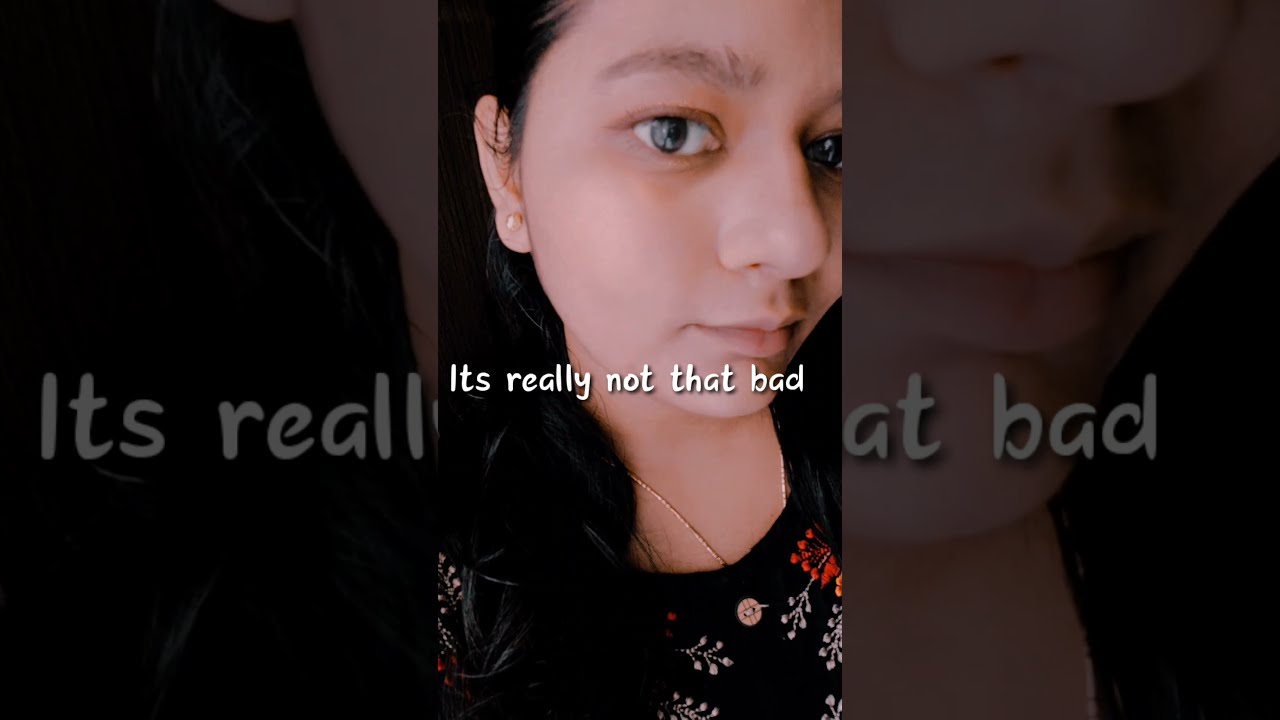The image is a close-up shot, possibly a screen grab from a TikTok video, featuring a young girl who appears to be around 17 years old. She has long black hair cascading past her shoulders, and she wears a thin gold necklace along with light peach pearl earring studs. Her attire is a black blouse adorned with white and red floral patterns and features buttons, suggesting it might be a cardigan or a similarly styled top. The girl exhibits big brown eyes and a light brown complexion, with a somber and serious expression directed at the camera. Text in white lettering overlays the image, stating, "it's really not that bad." The picture is presented in high quality and measures eight inches wide by five inches tall. The backdrop and her clothing's predominant black hue create a dark overall color scheme.